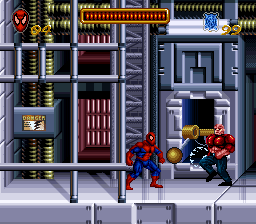This image is a detailed screenshot from a Spider-Man video game. In the upper left-hand corner, there's an icon of Spider-Man's mask, depicted with a red face and lighter-colored red eyes, accompanied by the number "04" in gold, signifying the player's number of lives. In the upper right-hand corner, a blue web icon displays the number "99". The top section of the screen features a gold bar marked with numerous vertical red hash lines, likely indicating the character’s health status.

The setting is a gray metallic surface, resembling a high-tech or industrial area. The background reveals two yellow metal pipes; one runs vertically along the left side, while the other runs horizontally at the top. These pipes have small black rings adorning them. Adjacent to the pipes, there’s a high-voltage danger electrical box fitted with gold-colored coils. Additionally, the backdrop includes a large metal square, a metal ladder-like object, and a red area near a doorway on the right side of the ladder structure.

In the foreground, there are several metal poles: two vertical and three horizontal, with some horizontal poles resembling a section of a ladder. Spider-Man, dressed in his iconic red and blue outfit, stands in the middle right of the frame. Facing him is a red, muscular character wearing blue jeans, potentially a villain from the game. Between them lies a gold ball. The overall aesthetic is cartoony, consistent with the typical video game art style.